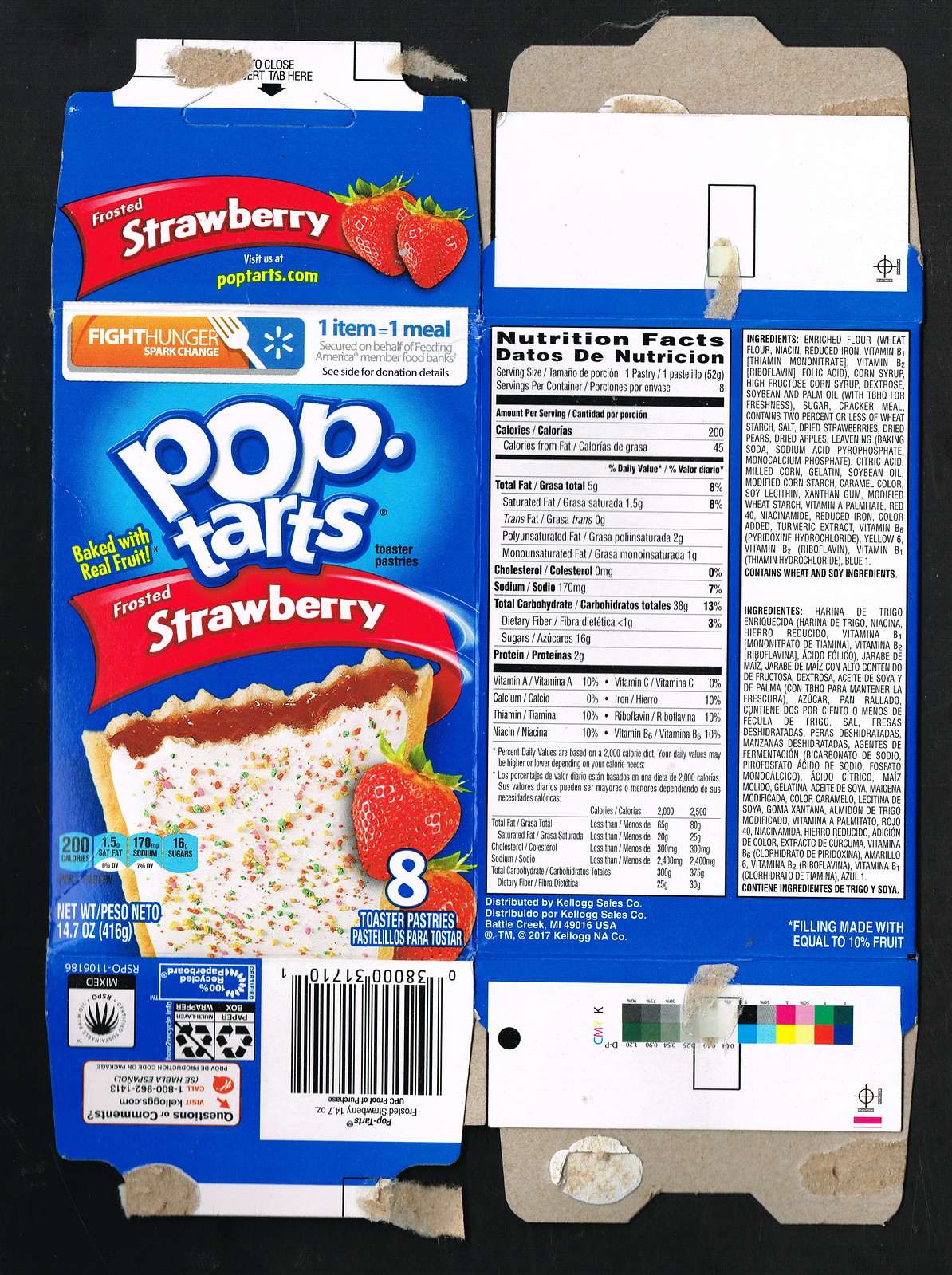This image depicts a partially flattened Kellogg's Pop-Tarts box, showcasing both the front and back. The featured flavor is Frosted Strawberry. On the front, the box prominently displays two vibrant images of strawberries below which the brand's website, "Pop-Tarts.com," is mentioned for more information. A notable collaboration between Pop-Tarts and Kellogg's to fight hunger is highlighted. Dominating the front cover, the Pop-Tarts logo appears in bold white and blue bubble letters. Just below, an appetizing illustration of a frosted strawberry Pop-Tart is shown with its top broken off, revealing the rich strawberry filling. The Pop-Tart is adorned with colorful sprinkles over a layer of white icing. The packaging indicates that there are eight pastries per pack. The bottom of the box features a visible barcode.